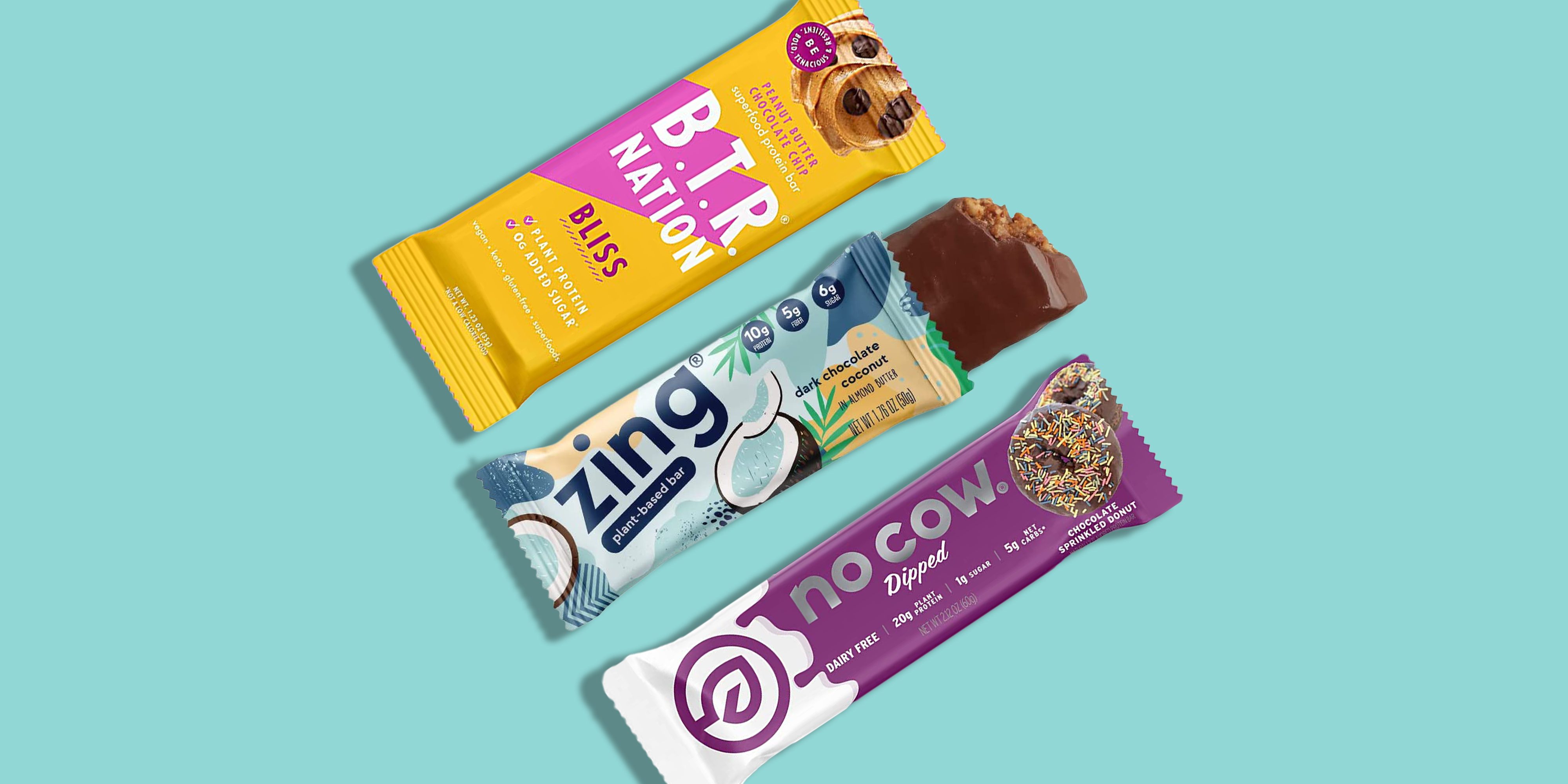This horizontally aligned rectangular image features a pretty light green background without any borders or text. Arranged diagonally, three different nutrition bars are stacked on top of one another. At the top, the unopened BTR NATION bar sits in a predominantly yellow package with "BTR NATION" written in white, all-caps letters, and "BLISS" beneath it. In the middle, the ZING bar, with its blue and green patterned label, is partially opened to reveal its dark chocolate and crispy center. The ZING bar prominently displays "Dark Chocolate Coconut" as the flavor and features small circles indicating nutritional details that are too small to read. The bottom, unopened bar is from No Cow, wrapped in purple and white packaging. It has "No Cow" in gray text followed by "dipped" in white letters, and it showcases an image of a sprinkled donut.